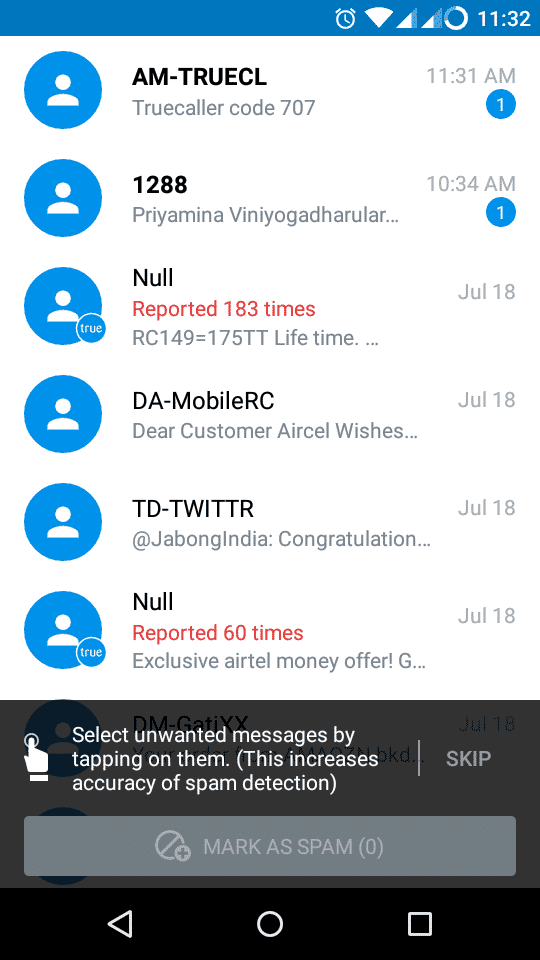This image is a screenshot from a mobile phone displaying a mobile messaging application. At the very top of the screen, there's a blue status bar featuring several icons: an alarm logo, the Wi-Fi signal indicator, two sets of signal bars, a battery logo, and the time displayed as 11:32 on the far right.

Below this blue stripe, there is a list of messages, clearly indicating that this is a message inbox page. The messages are as follows:
1. A message from "am true CL" received at 11:31.
2. A message from "1288" received at 10:34.
3. A message labeled "null reported 183 times" with a date stamp of July 18th.
4. A message from "da mobile RC," also dated July 18th.
5. A message from "TD Twitter" dated July 18th.
6. Another "null reported 60 times" message dated July 18th.

At the very bottom of the screen, there is a black field with white text instructing the user to "Select unwanted messages by tapping on them. This increases accuracy of spam detection." Directly beneath this informative text is a gray button with white text labeled "Mark as spam."